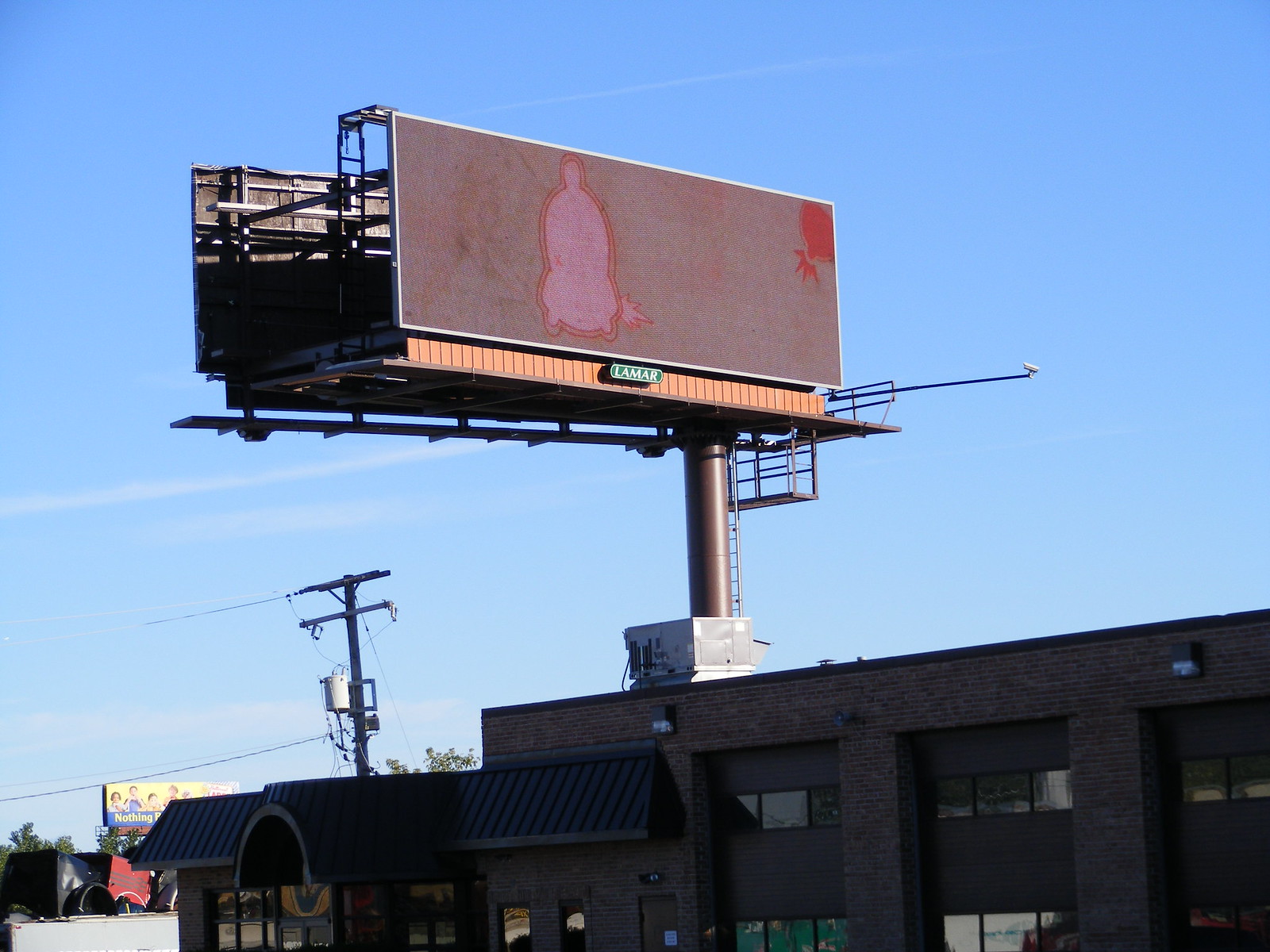In the contemporary photograph, the focal point is a prominent, somewhat dilapidated billboard situated almost centrally towards the top of the frame. The billboard, which appears aged and dirty, features faint, indistinct imagery with hints of red. A ladder used by billboard changers is visible, extending up to a platform in front of the billboard. Supporting this structure is a substantial post. 

Behind the billboard, power lines stretch across the scene, connected to a power pole equipped with a transformer. In front of the billboard stands a two-story building, identifiable by its various doors and windows suggesting it is likely a storefront. An air conditioning unit is perched atop this building. 

The sky above is a strikingly bright blue, adding a vibrant backdrop to the image. Finally, in the distance, specifically on the lower left-hand side, a second billboard is visible, further adding to the urban atmosphere of the scene.